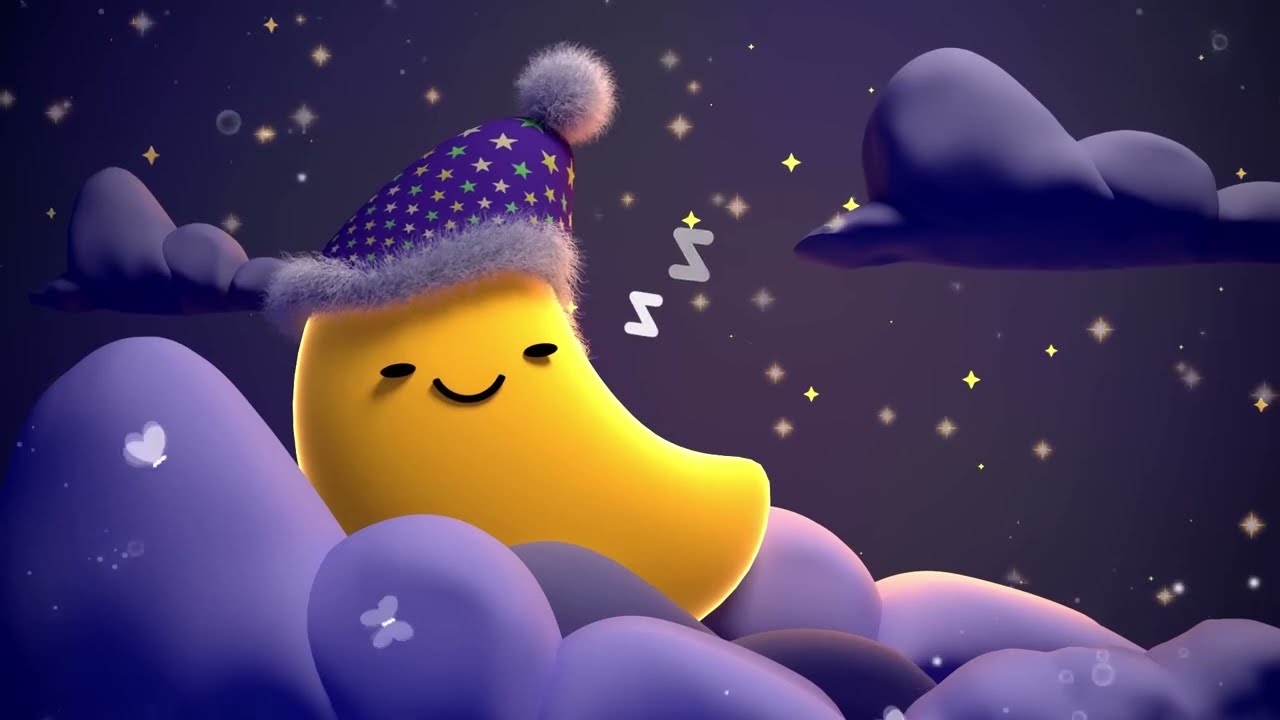This 3D-rendered, animated image showcases a chubby, crescent-shaped yellow moon nestled comfortably on fluffy purple clouds. The moon, which sports a cheerful smile and protruding eyes casting shadows, wears a cozy purple nightcap adorned with yellow and blue stars, complete with a fluffy base and a pom-pom on top. Two white 'Z' letters float above its head, indicating it is asleep. In the foreground, delicate moths or butterflies flutter around the clouds. The scene is set against a dark, star-studded sky with a mixture of yellow and purple stars, and a dark cloud looms in the right corner, adding depth to the dreamy atmosphere.